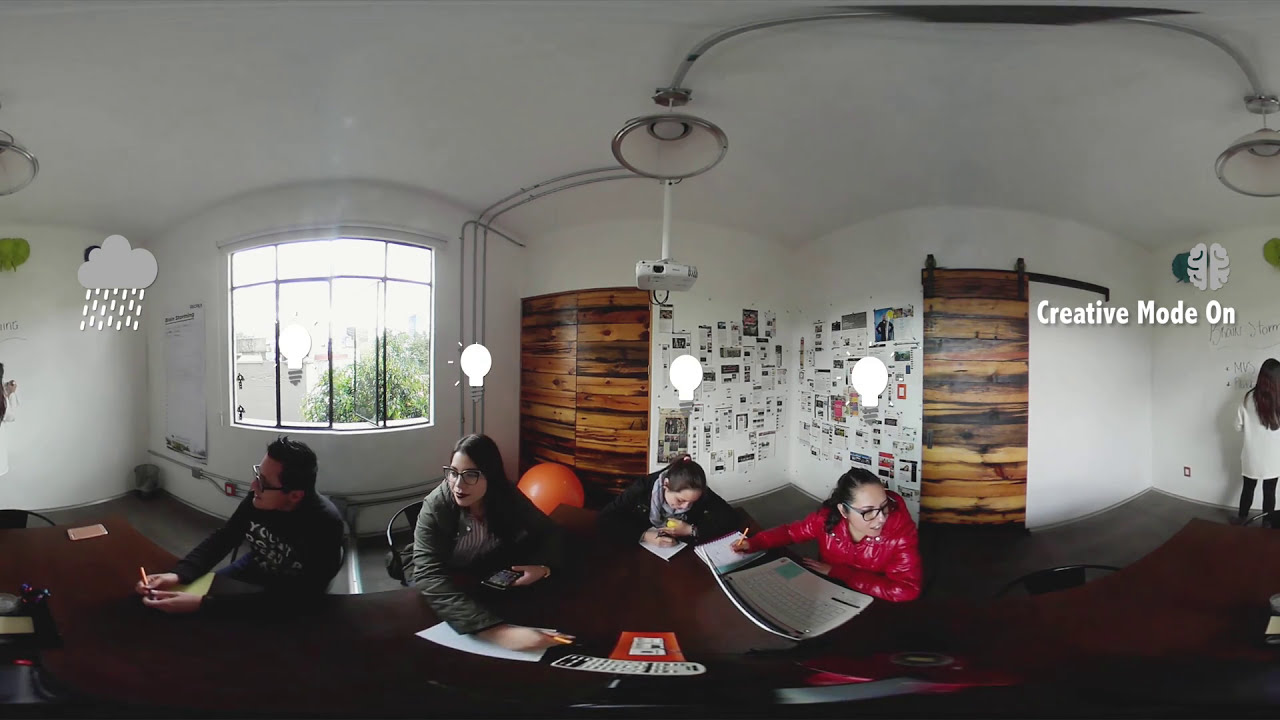The image portrays an indoor office studio space with a long table at which four young individuals, appearing to be in their late teens or early twenties, are seated and engaged in various activities. On the left, a man in a sweatshirt and glasses sits next to a woman with long black hair and glasses. Next to her is another woman with a ponytail and scarf, looking down and writing on a notepad. To the far right, a woman in a bright red coat with black glasses works on a laptop. Animations have been added to the picture, with light bulbs over the heads of the three women in the center, suggesting moments of inspiration. A text saying "Creative Mode On" accompanied by a brain graphic is superimposed on the right side, while a rain cloud graphic is positioned on the left. A woman can be seen working at a whiteboard at the extreme left of the panoramic scene. The room has white walls with a montage of photos in one corner and large windows letting in natural light, revealing a tree and a building outside. The doors are sliding, moving along a rail rather than on hinges. The overall ambiance suggests a creative and collaborative environment.